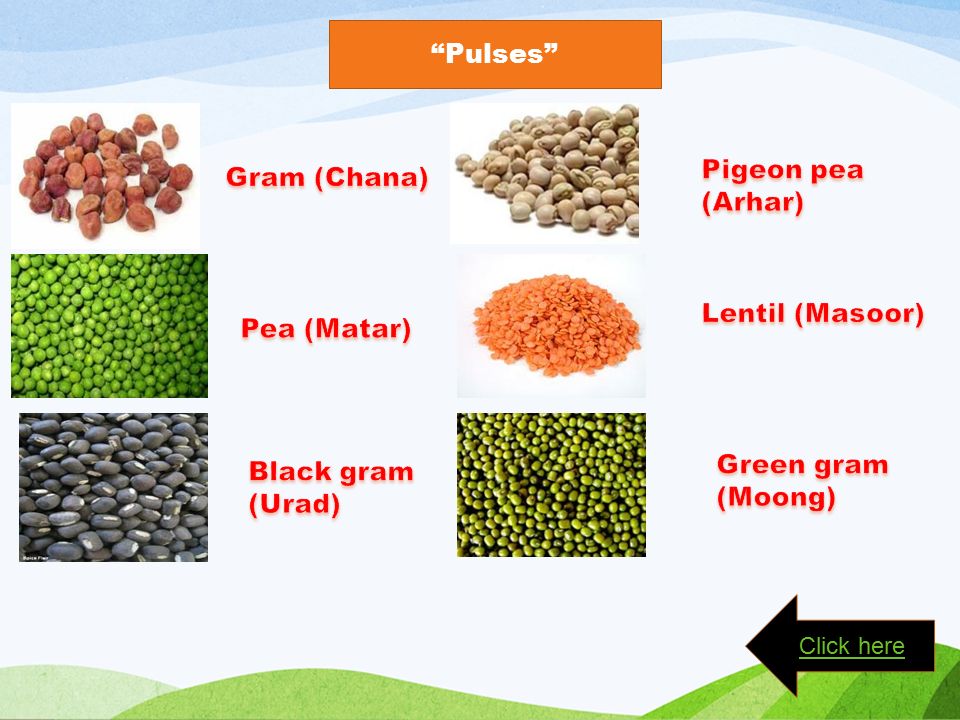The image is an informational diagram showcasing various kinds of pulses. At the top center, inside an orange rectangular box, the word "PULSES" is prominently displayed in white and in quotation marks. Below this heading, the image is divided into two columns, each featuring three different types of pulses along with their images and names. 

On the left column:
1. At the top, there is Gram (Chana).
2. Below that, there is P (Matar).
3. At the bottom, there is Black Gram (Urad).

On the right column:
1. At the top, there is Pigeon Pea (Arhar).
2. Below that, there is Lentil (Masoor).
3. At the bottom, there is Green Gram (Moong).

The names of the pulses are clearly labeled with their common names followed by their regional names in parentheses. Each pulse type is represented with an accompanying image to visually depict its appearance. The background of the image features blue and green wavy patterns, adding a visual appeal to the information. At the bottom right corner of the image, there is an arrow pointing left with the words "CLICK HERE," indicating a call to action.